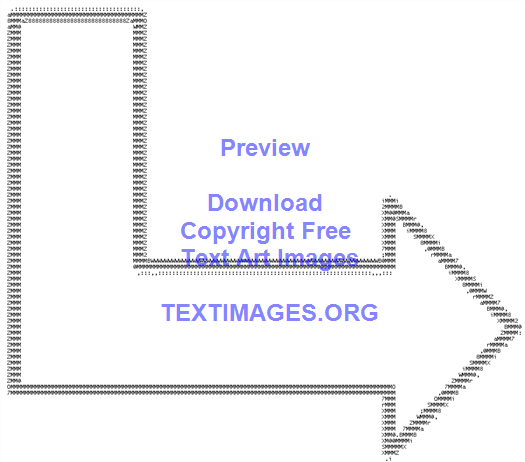The image features an L-shaped arrow that starts at the top left, curves downward, and then points to the right. This arrow is not drawn but meticulously crafted using characters from a typewriter or keyboard, creating a detailed text art image on a white background. Superimposed on this intricate arrow are blue-purple words that read "Preview," "Download," "Copyright Free," and "Text Art Images." In the upper right quadrant, and within the arrow itself, the text "TEXTIMAGES.ORG" is prominently displayed, advertising the website where such text art images can be found.